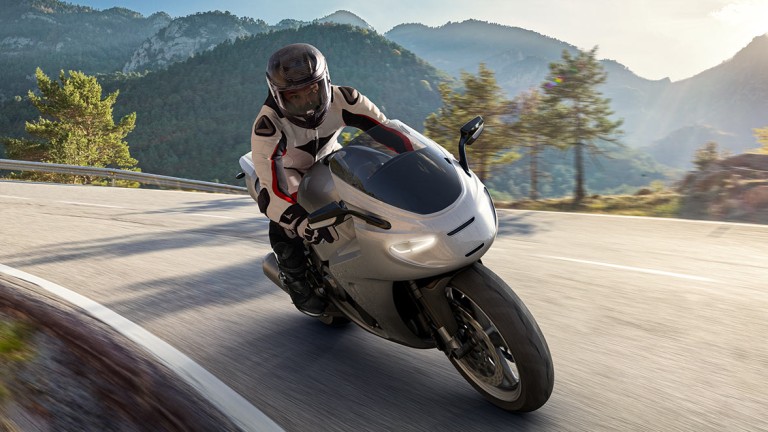In this vibrant action shot, a motorcyclist on a sporty, silver motorcycle is captured speeding down a concrete road in a mountainous area. The rider is hunched over the handlebars, clad in a white leather jacket adorned with navy, black, and red patches, and a black helmet with the face shield down for protection. The motorcycle, with its white front, black tires, large visor, and reflective rearview mirrors, is central in the image, angled towards the bottom right corner as if moving at high speed. The lush backdrop features green tree-covered mountains with snow-tipped peaks, a bright sunny sky casting light over the scene, and blurred elements that enhance the sense of motion. The colors spotted include whites, reds, blacks, greens, light blue, and grays, all contributing to the dynamic visual narrative of a thrilling motorcycle journey through a picturesque, mountainous landscape.